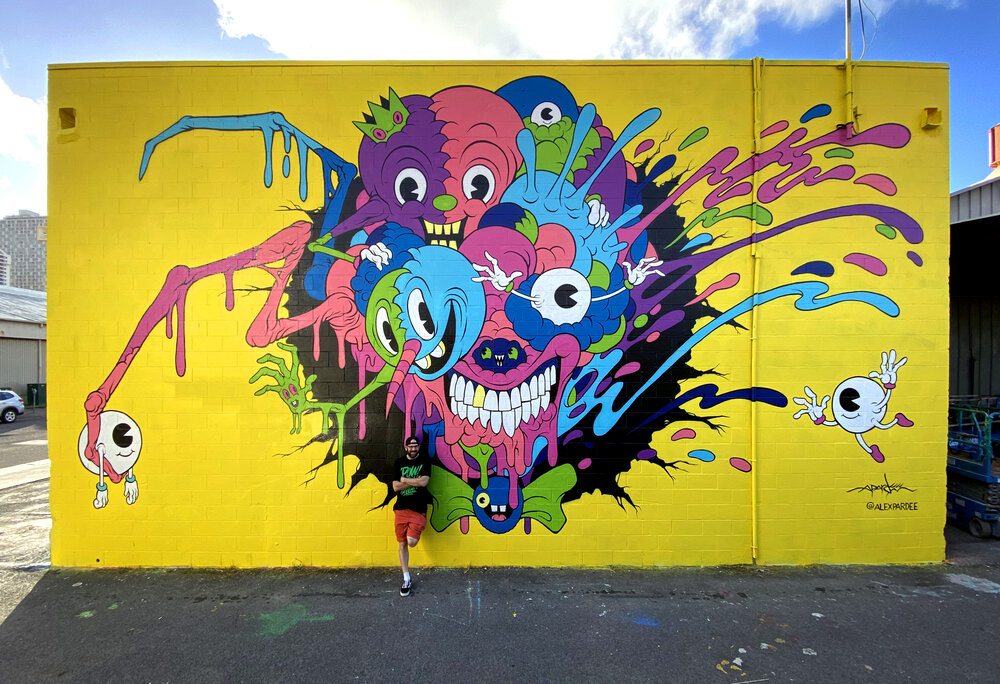The image showcases a large, abstract mural painted on a brick wall of a building, which can be seen against a clear blue sky with a few clouds suggesting a sunny day. The mural, set against a vibrant yellow background, features a colorful and whimsical array of cartoon-like monsters and faces with tentacle-like extensions reaching towards small Pac-Man-like figures. The bright colors used include purples, pinks, blues, greens, and some whites, with black details accentuating the background. One eye-catching element of the mural is a large, grinning face displaying a set of teeth, one of which is distinctly yellow. Leaning against the mural is a young man, possibly the artist, dressed in a black baseball cap worn backwards, a black T-shirt with green writing, and orange shorts. He poses with one leg propped against the wall and the other on the cement ground. The detailed and playful nature of the mural's design, combined with the vibrant color palette, suggests a comical or surreal artistic intent.